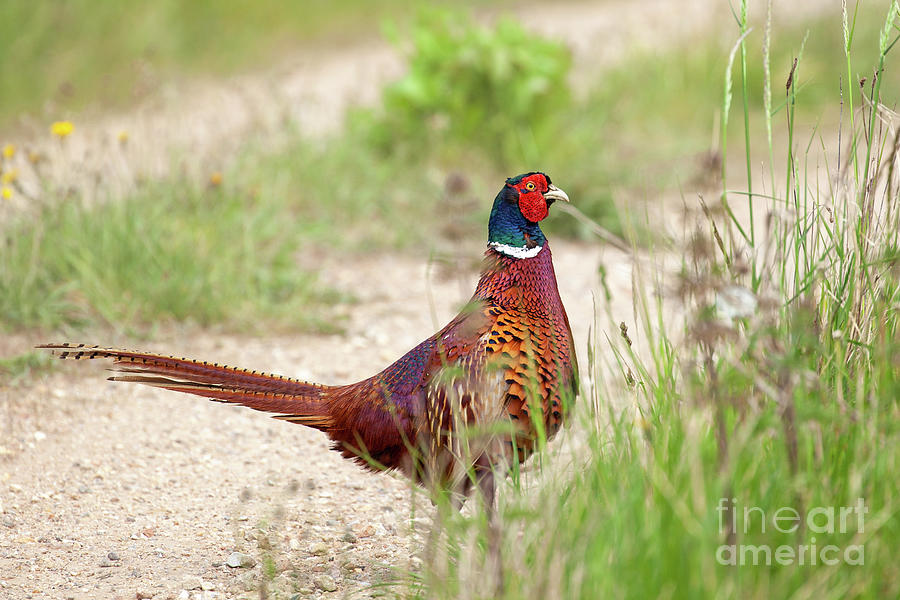The image depicts a vibrant pheasant standing centrally on a dusty, rock-strewn pathway that is flanked by tall grasses and scattered yellow flowers. The bird, reminiscent of a colorful rooster, features a striking array of feathers: its back displays a purplish sheen, while its wings are adorned with white stripes. The chest feathers range from golden to black, with a copper hue on the lower part of its neck, which is separated by a white strip from the deep blue and slightly green feathers around its beak and head. Notably, the pheasant has a noticeable red patch around its yellow eyes and a white beak. It boasts a long, copper-colored tail. The overall setting is outside, evoking a rustic, natural scene with the bird positioned towards the right, accompanied by text in the bottom right corner reading "Fine Art America."